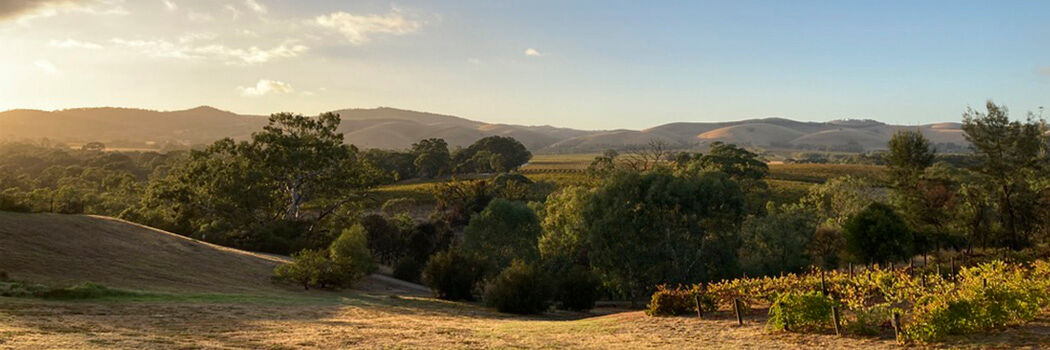This panoramic landscape photograph, taken from a rectangular perspective, showcases a vast valley with rolling hills blanketed in green and yellow grasses. The vibrant scene is dotted with numerous trees adorned with lush green leaves. In the bottom right corner, neat rows of green, bushy cultivated crops—possibly a vineyard—are bordered by wooden pillars and wire trellises. The expansive sky overhead changes from light blue on the right to a warm, yellowish hue on the left, suggesting a sunset or sunrise. A clear path weaves through the scene, casting a shadow on its left side, perhaps from an unseen tree. Distant mountains lend depth to the background, appearing slightly faded and foggy under the mostly clear sky, punctuated by occasional clouds. This serene and detailed depiction reveals the natural beauty of a warm climate landscape, possibly reminiscent of southern France or another temperate region in Europe.